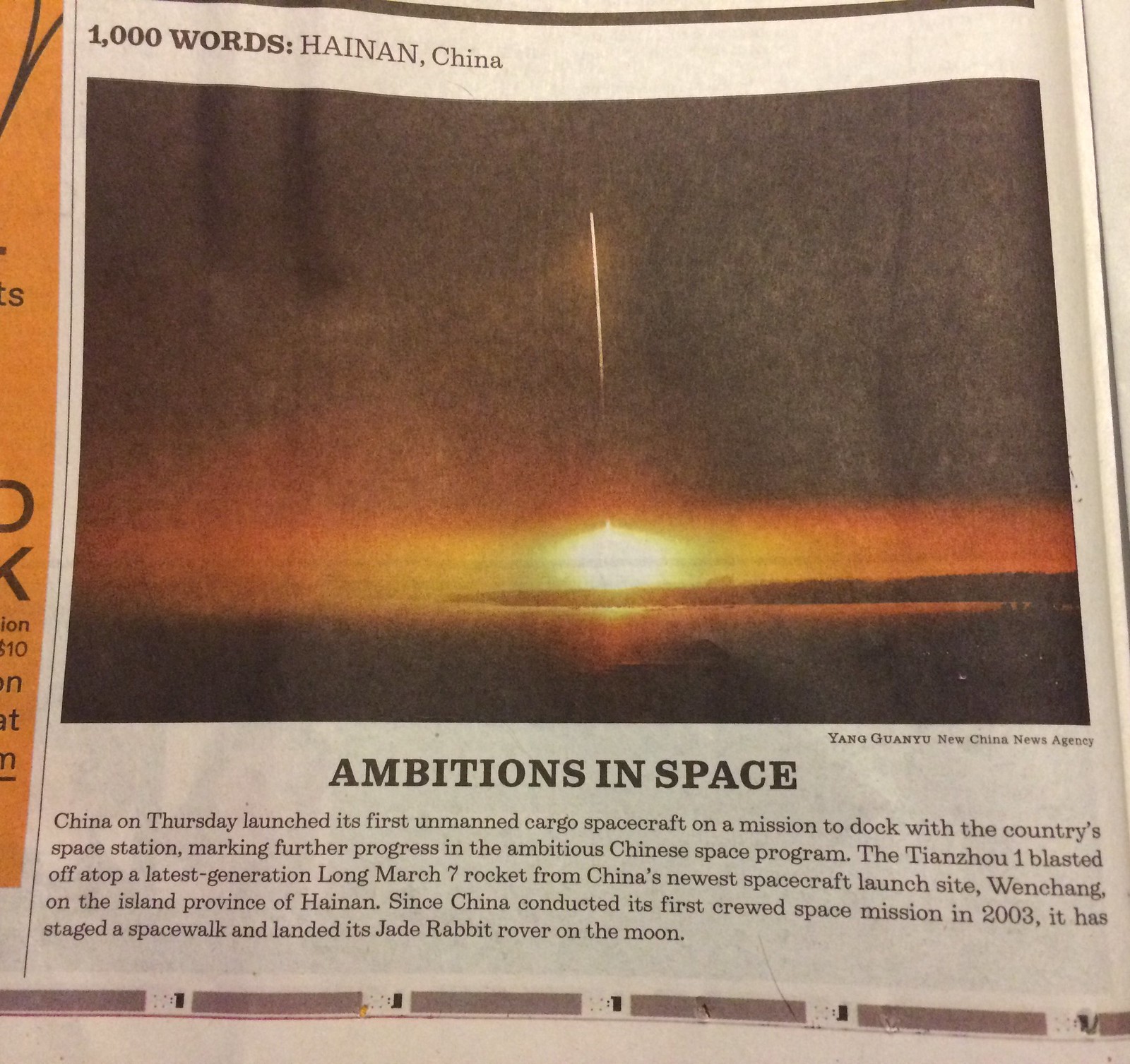The image is of a newspaper article titled "Ambitions in Space," featuring a photograph of a rocket taking off in the morning from China's newest spacecraft launch site in Wenchang, on the island province of Hainan. The rocket, Tianzhou-1, illuminated the bottom of the picture with a red glow as it ascended into the night sky atop a latest-generation Long March 7 rocket. The upper left-hand corner of the newspaper article shows "1,000 words, Hainan, China" above the photograph. The text beneath the title details that China launched its first unmanned cargo spacecraft on a mission to dock with the country's space station, marking significant progress in the Chinese space program. China's ambitious space endeavors have included its first crewed space mission in 2003, a spacewalk, and the landing of the Jade Rabbit rover on the moon.